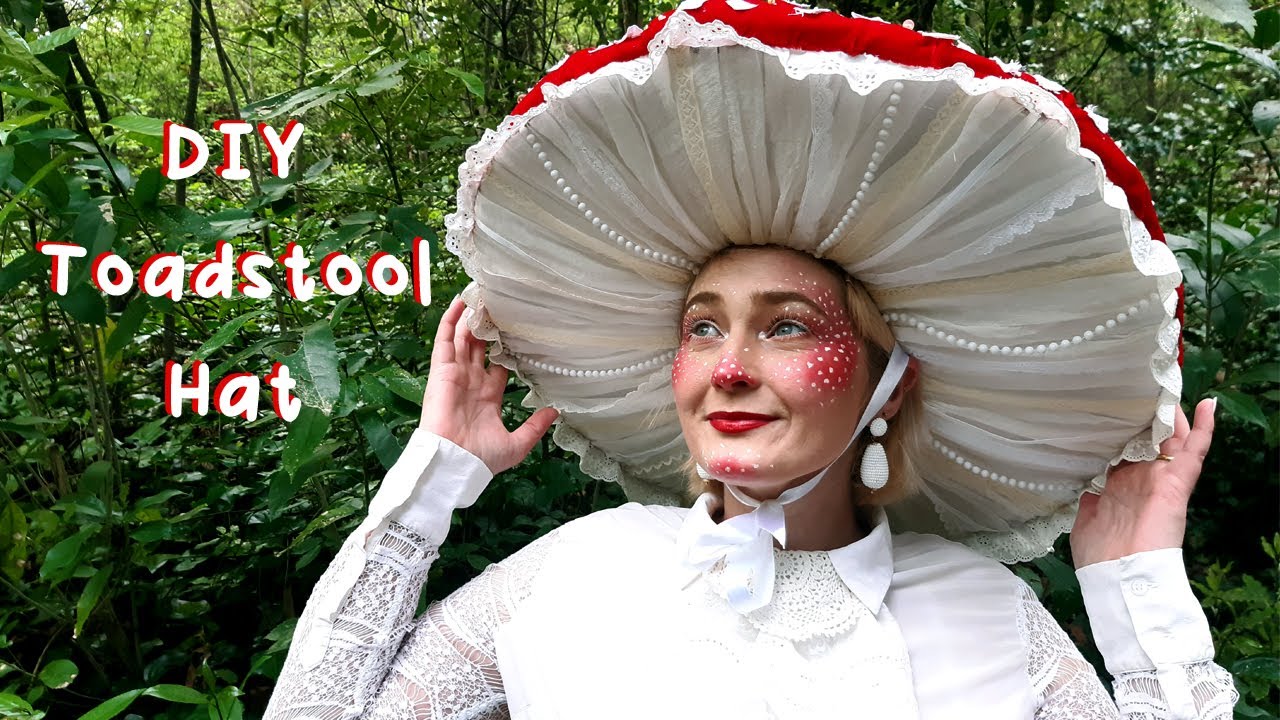The image showcases a young woman standing in a lush green forest, wearing an elaborate, oversized toadstool hat that is about three times the size of her head. The hat features a frilly white fabric undersurface adorned with rows of pearl beads arranged in sections, and the top is red with white spots, mimicking the appearance of a classic toadstool. The woman sports distinctive makeup, including red blush with white spots on her nose, cheeks, and chin, complemented by red lipstick. She is dressed in a white top with lace around the high collar and sleeves, further enhancing the whimsical aesthetic. The photograph includes white text with a red border, arranged in three lines that read "DIY Toadstool Hat," suggesting it may be a thumbnail for a YouTube video or a website article. This upbeat and detailed composite illustration contrasts the vibrant hat and makeup against the serene green background, making the DIY theme clear.